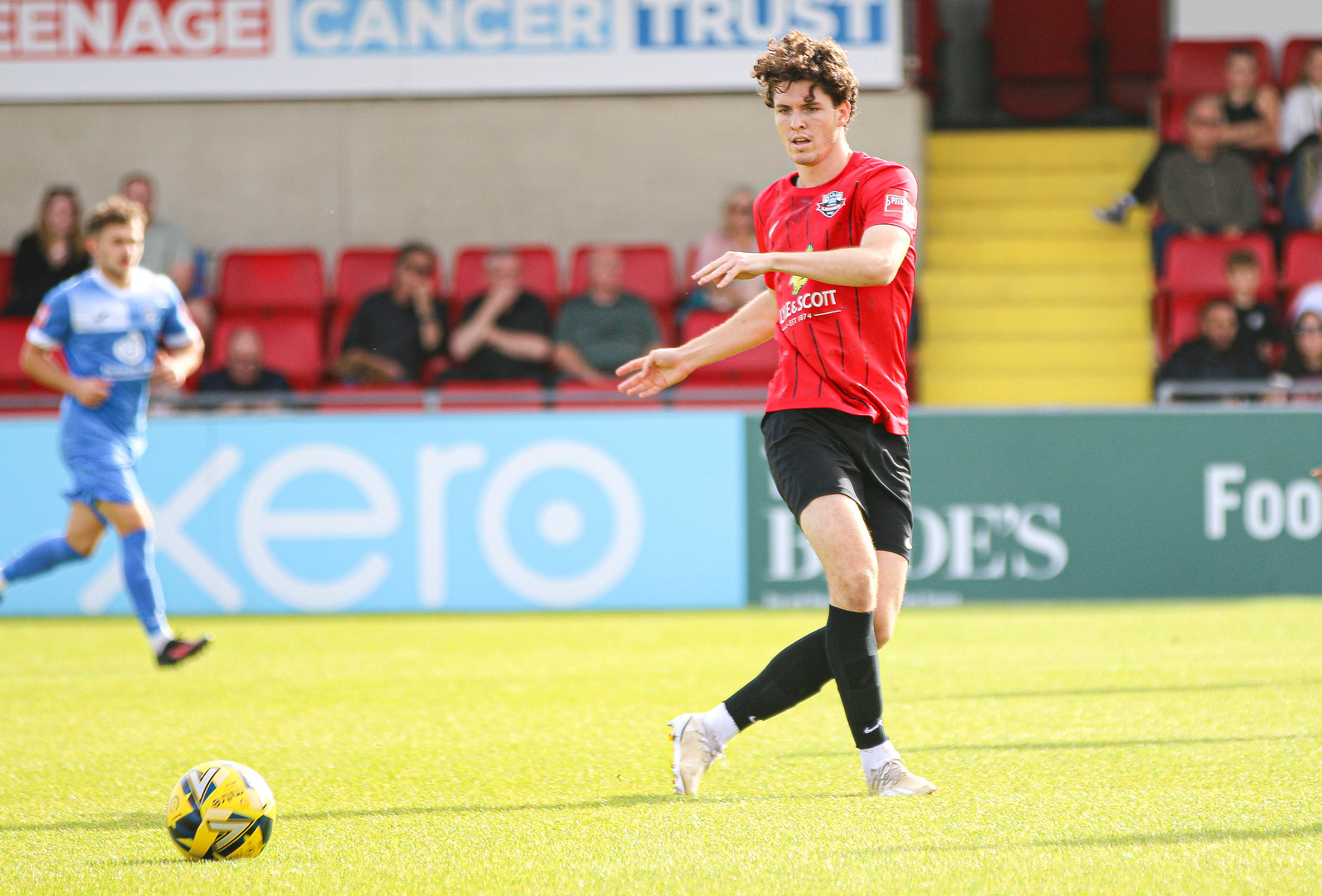The image captures an intense moment in a soccer game on a lush green field. Central to the photograph is a white soccer player with brown hair, donning a red jersey, black shorts, black shin pads, and white sneakers, appearing to have just kicked a yellow and black soccer ball. To the left in the background stands another player, a white man in motion, dressed entirely in blue — shirt, shorts, and shin pads. The stadium behind them features red seats and yellow stairs leading up from the seats. Spectators, though not densely packed, are visible, keenly watching the game. Above the seating, the signage reads "Teenage Cancer Trust," accompanied by advertisements below the seats displaying "XERO," followed by partial letters "B O E S" and "F O O."